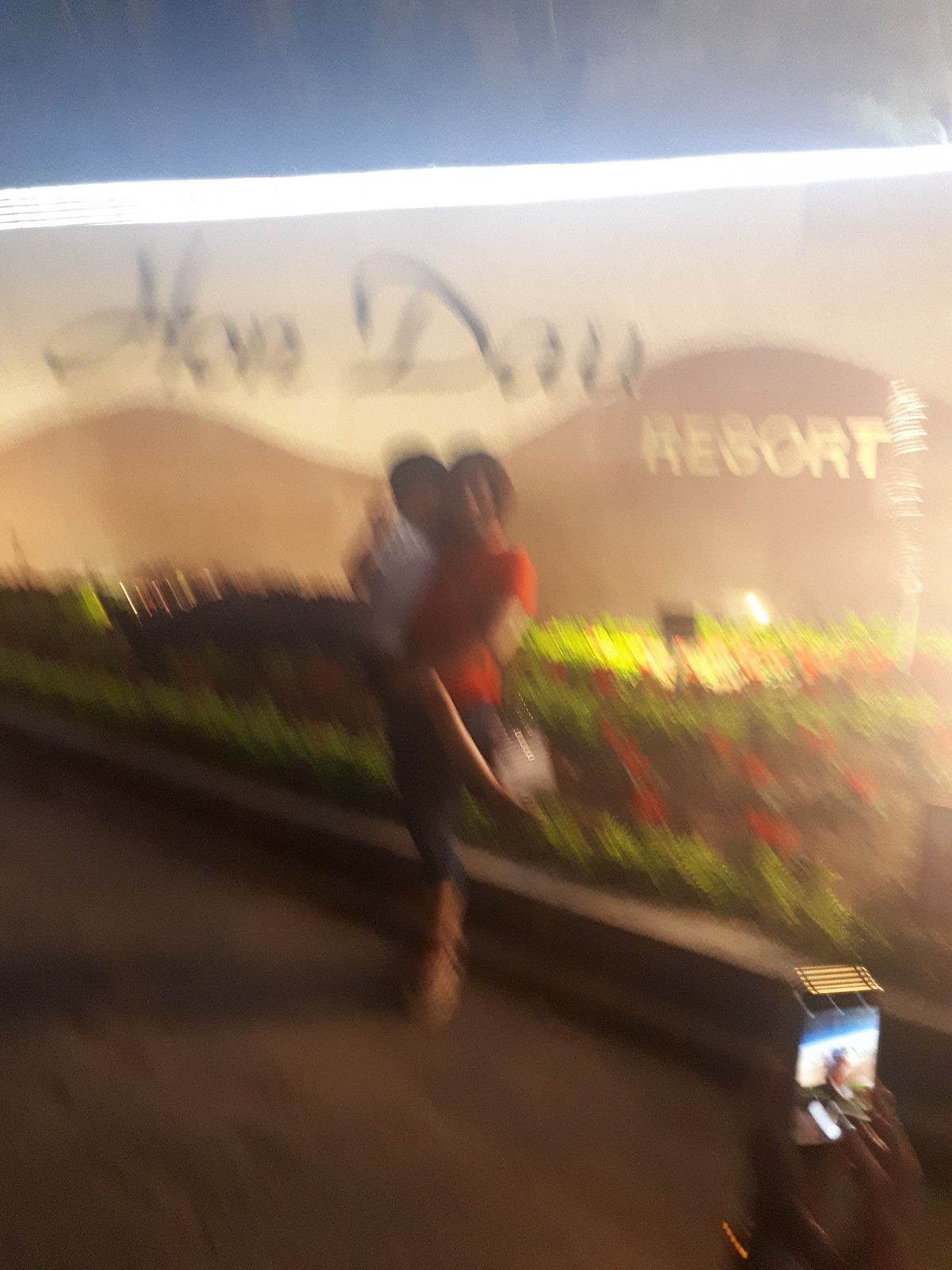In this blurry outdoor photograph, a woman with short dark hair is holding what appears to be a child, estimated to be around six or seven years old, though possibly younger. The woman is dressed in a red shirt, capri pants, and sandals. The child, whose long legs are noticeable despite the blur, adds to the sense of their taller stature. They are standing in front of a sign, partially obscured by the blur, which seems to read something related to a resort and features an image of a mountain. The base of the sign is surrounded by a vibrant bed of flowers, displaying bright hues of red, yellow, and green. The background and setting, though indistinct, suggest a cheerful, welcoming environment.